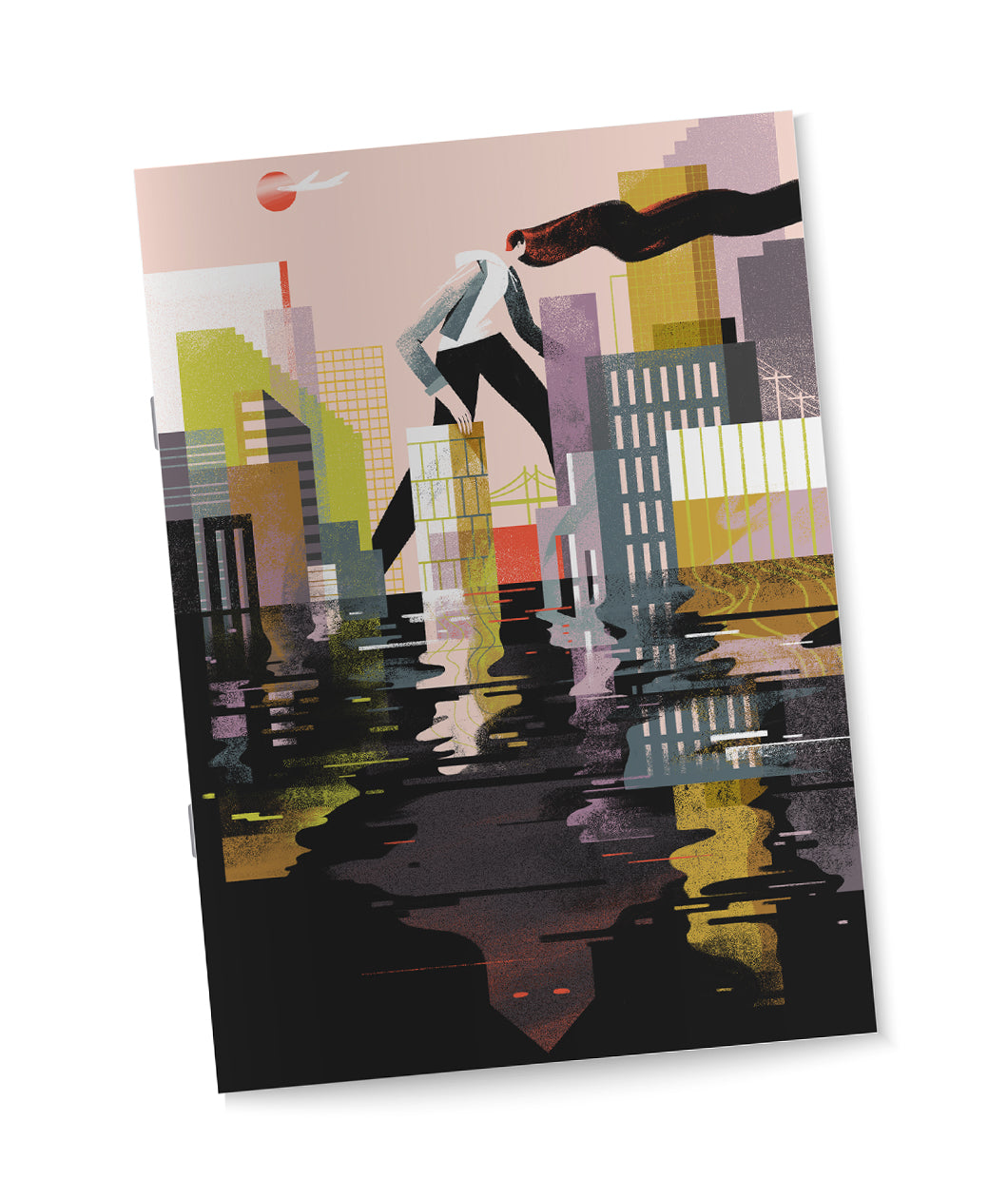This piece of abstract modern art stands against a white background and is slightly tilted to the left. The composition features a dramatically divided scene, split into two distinct halves. The bottom half of the painting is dominated by an ominous pool of black liquid, which may suggest water, with a small yellow stone submerged within it. Hovering above, the top half of the painting is filled with a stylized cityscape composed of high-rise buildings in hues of yellow, purple, gray, and umber. 

Towering over this cityscape is a disproportionately tall and imposing figure of a woman, characterized by flowing long hair that streams off to the right. Her attire appears to be a mix of a white shirt, a gray hoodie with hints of pink, and black pants. Between her legs, there is also a glimpse of a suspension bridge in the distant background. 

Further enriching the surreal atmosphere, in the upper left corner, there’s a small red dot—a sun or a moon—with a wisp of a white cloud partially obscuring it. The sky takes on a pinkish hue, adding to the dreamlike quality of the scene.

In the black pool below, mysterious red eyes peer out, contributing to the enigmatic and slightly sinister mood of the composition. Overall, the artwork blends elements of art deco and anime styles, presenting a cityscape that is both half-drowned and eerily haunting, encapsulating a sense of foreboding and otherworldliness.